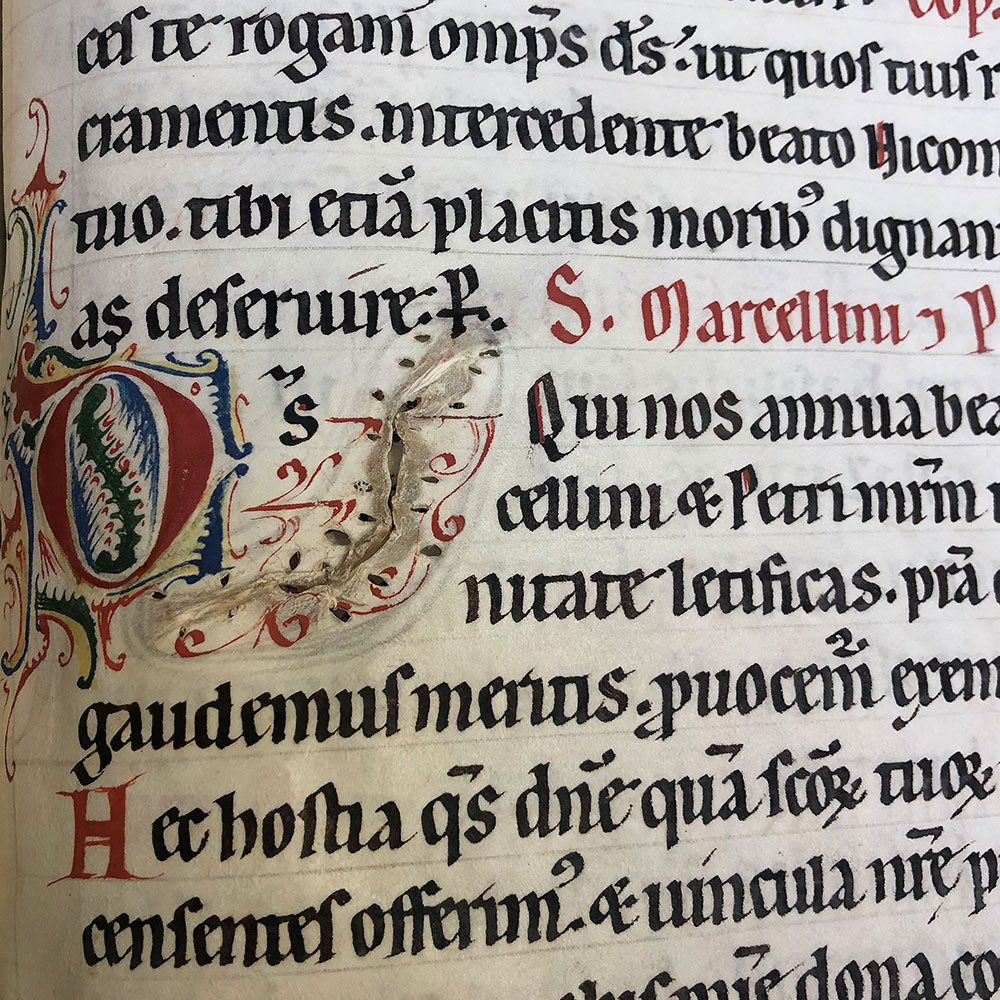This image captures a close-up view of a medieval manuscript, possibly dating between 1225 and 1275, potentially from Austria. The page features ornate calligraphy in a non-English language, likely Latin or Italian. The script consists of ten lines of black ink with occasional red lettering that appears to include the name "S. Marcellum" and letters "S," "M," "P," and "H." On an off-white paper background, the text is punctuated by a large decorative design on the left side, resembling a grand, ornate letter "O" with a blue center. Surrounding this letter is an intricate illustration featuring gold, red, blue, and green hues, possibly incorporating elements that look like a peacock feather or a spine. The overall impression is one of historical richness and artistic detail, indicative of the manuscript's sacred or scholarly importance.